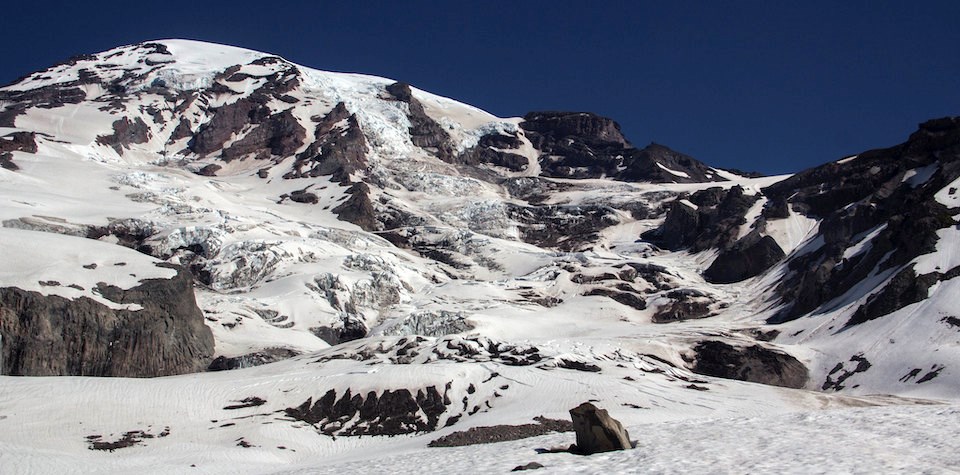The photograph captures a breathtaking mountainous region under twilight with deep, almost purple-blue hues enveloping the sky. The tallest mountain stands at the upper left of the image, its slopes gradually descending to the right yet never dipping below a quarter of the frame. Snow and ice blanket most of the landscape, with more accumulation on the shadowed, left side of the mountain, while the sun-exposed right side shows less snow cover. The rugged peaks reveal patches of bare rock amidst the snow, with some rocky outcroppings completely devoid of snow due to windswept areas. The foreground includes a mix of snowy surfaces and exposed rocks, indicative of a windswept environment. The scene is devoid of any human presence, emphasizing the pristine and untouched nature of this tranquil high-altitude wilderness.